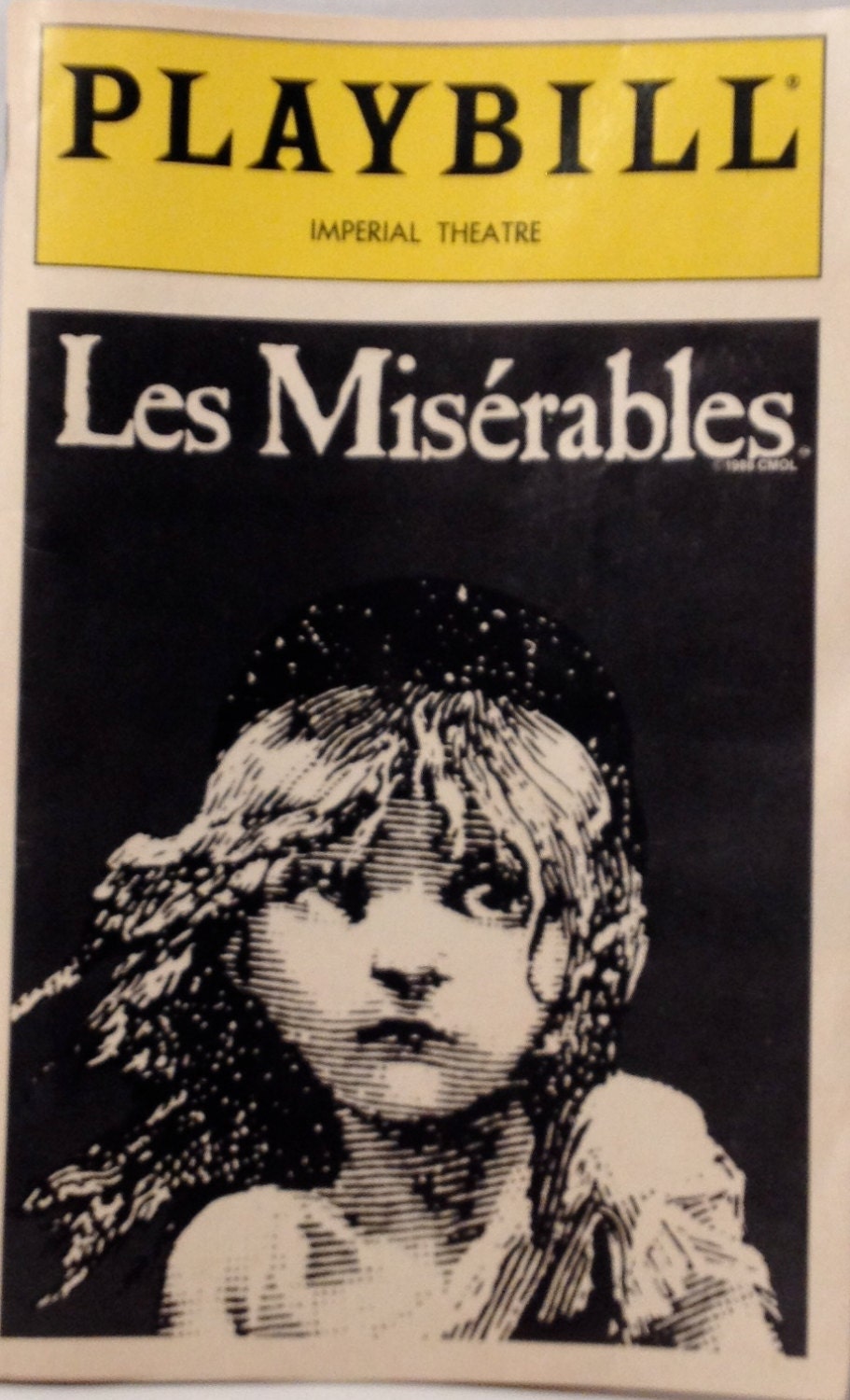This image is a detailed picture of a Playbill cover for the Broadway musical *Les Misérables* at the Imperial Theatre. At the very top, a yellow background frames the bold black text "Playbill," followed by "Imperial Theatre" in smaller, black print. Below this header, the cover features a prominent black background showcasing "Les Misérables" in striking white text. Central to the design is the iconic, haunting illustration of a young, destitute girl. She has long, light-colored, slightly unkempt hair blowing gently from right to left. Her dark, expressive eyes convey a sense of vulnerability and fear. She attires a tattered white dress, with one shoulder partially uncovered, encapsulating the poignant imagery associated with the production.